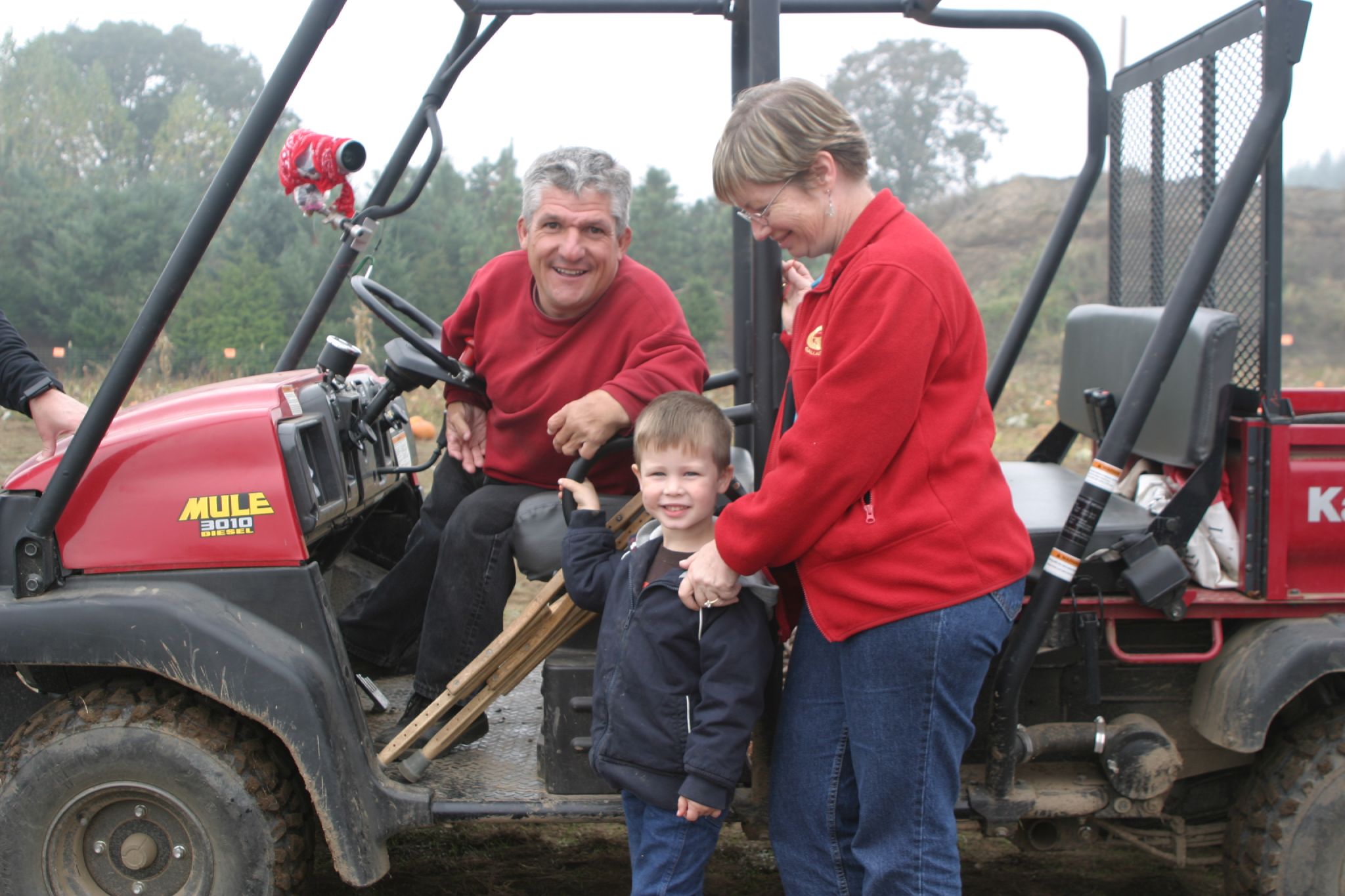In the photograph, Matt Roll is behind the steering wheel of a red tractor with a black frame, smiling as he sits in the driver's seat. Standing in front of the tractor is a little boy with dirty blonde hair, dressed in a navy blue jacket and blue jeans, who appears to be holding onto the side of the tractor. Next to the boy is a woman, likely his grandmother, wearing a red fleece sweater jacket, blue jeans, and glasses, facing towards him with her left hand resting on his shoulder. The boy and Matt are both visibly happy, with smiles on their faces. In the background, there are numerous trees and a big dirt pile on the right side of the image, while the sky above is white, indicating it's daytime. A partially visible hand, presumably another family member's, is touching the top front of the tractor, where a camera or some device is positioned near the steering wheel. The family, comprising Caucasian members with fair to light skin, shares a moment of joy, surrounded by nature.